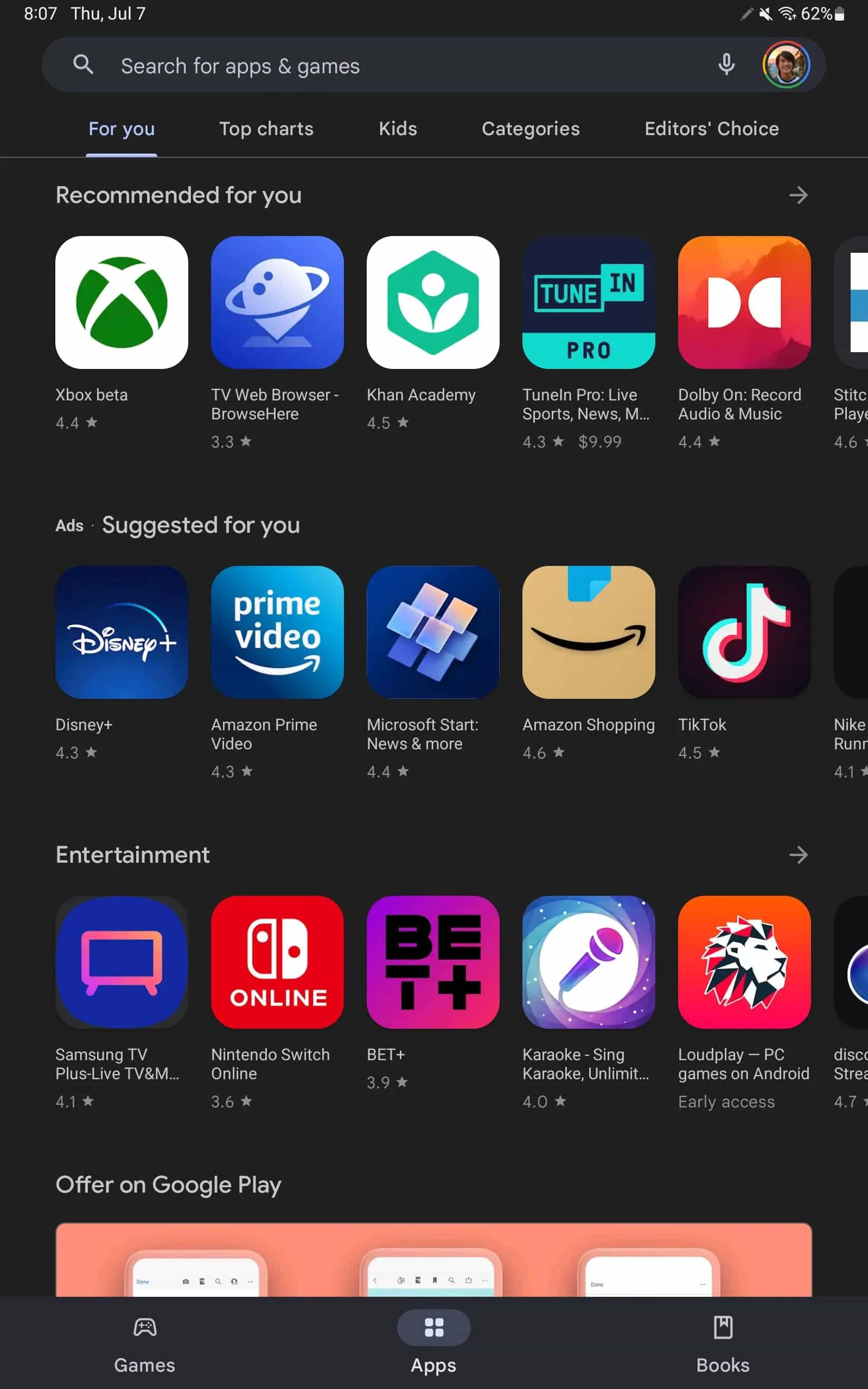The image showcases a digital interface against a black background. The top section displays the time as 8:07 on Thursday, July 7th, along with a battery level of 67%. Below this, there is a search box and a circular, multicolored icon with a person's picture inside it. The navigation options include "For You" which is underlined, "Top Charts," "Kids," "Categories," and "Editor's Choice."

A series of app icons appear beneath these categories. The visible icons include Xbox Beta, TV, Web Browser, Khan Academy, TuneIn Pro Live Sports, and Dolby On Record, followed by one that is partially cut off. 

Following these, there is a section labeled "Ads Suggested For You," featuring more app icons: Disney, Amazon Prime, Microsoft Start News & More, Amazon Shopping, TikTok, and another obscured icon.

The "Entertainment" category shows apps like Samsung TV, Nintendo Switch Online, BET, Karaoke, Loud Play PC, and one partial icon. An offering on Google Play is highlighted with a red box containing three smaller white boxes inside it.

At the bottom of the screen, navigation tabs are displayed: "Games," "Apps," and "Books."